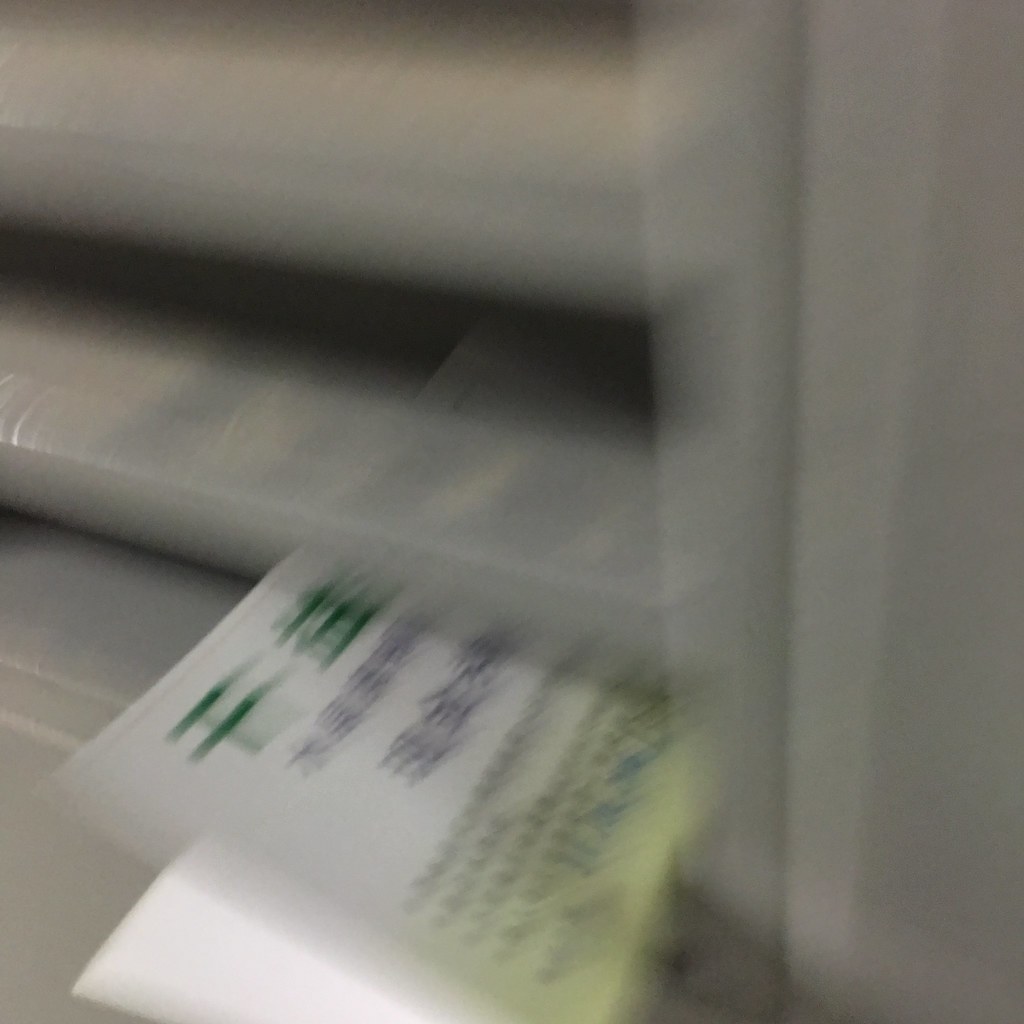The image is very blurry and out of focus, making it challenging to discern fine details. It features a gray background with horizontal black stripes, resembling a grate or a slot, potentially indicative of a mail slot, printer, or some sort of sorting apparatus. At the bottom of the picture, which is slightly more focused, a piece of paper is visible partially inserted into one of these slots. This paper has green Chinese characters at the top, followed by smaller black Chinese characters underneath. Below these, there is a light green section with more dark Chinese characters written on it. Some descriptions mention additional yellow and blue markings on the bottom part of the paper, possibly indicating a stamp or a seal. Overall, the setting could be reminiscent of an office window with bars separating staff from customers, or simply a mechanical device designed to handle documents.